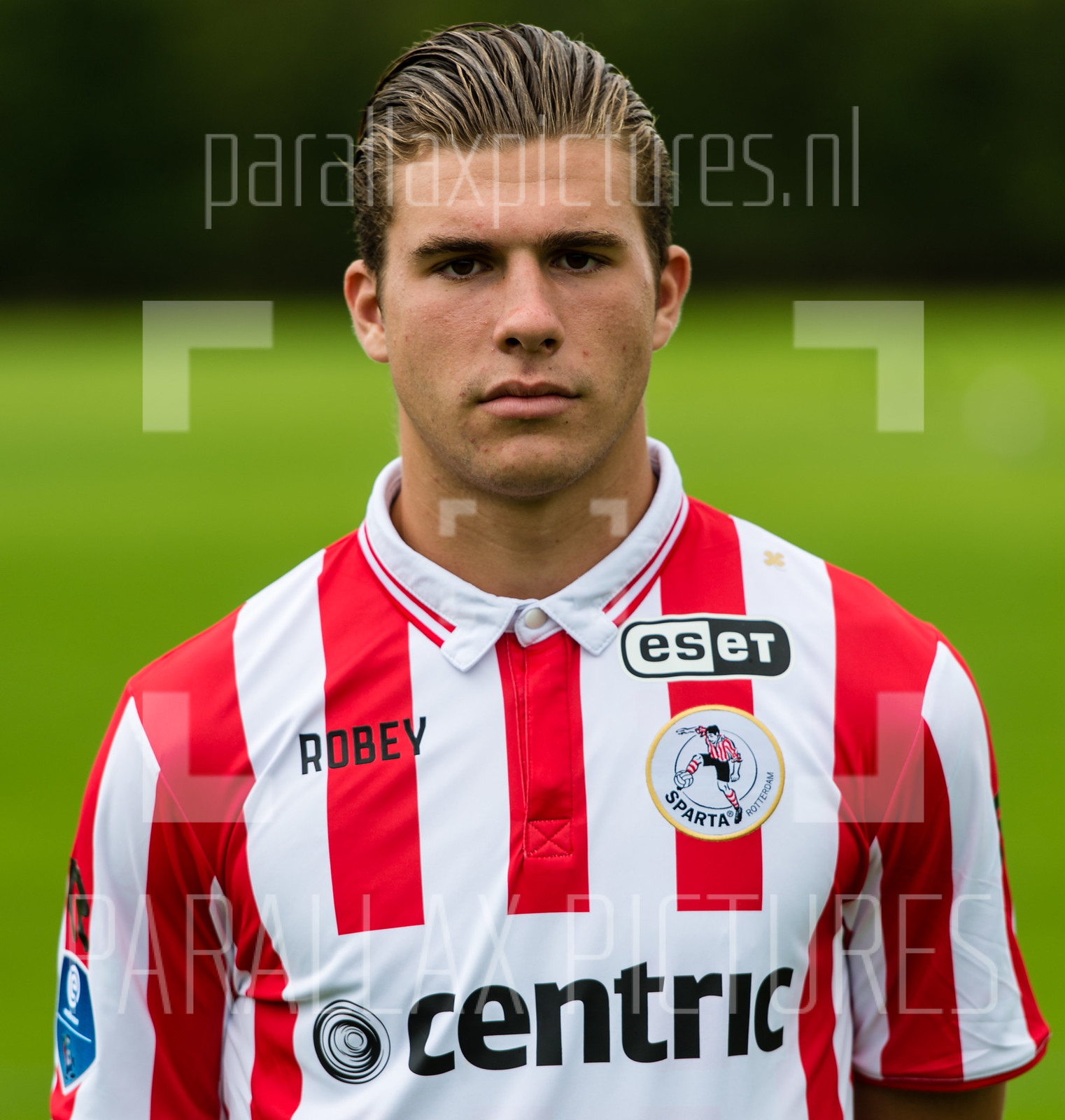The image features a young man in his 20s, who appears to be a soccer player, positioned prominently in the center. He has brown hair, which is slicked back, and he gazes directly at the camera with a serious expression. He is wearing a distinctive white jersey adorned with multiple red stripes, which run from the neck down to the chest, along the sides, and on the sleeves. The jersey is buttoned up all the way to the collar. 

At the center of the jersey, the word "CENTRIC" is printed in black letters. On the left side of his chest are two emblems: one reads "ESER" and features an illustration that seems to depict a person kicking a soccer ball. The other emblem, on the right side of his chest, reads "ROBEY." Above this, there's a patch with the words "Sparta Rotterdam," likely indicating his team. 

The background behind him is out of focus but appears to be a green soccer field, suggesting the photo was taken on or near a pitch. A faint watermark of "parallaxpictures.nl" runs across his forehead, indicating the source of the image. This detailed portrait seems to be a headshot, possibly intended for a team website or promotional material.